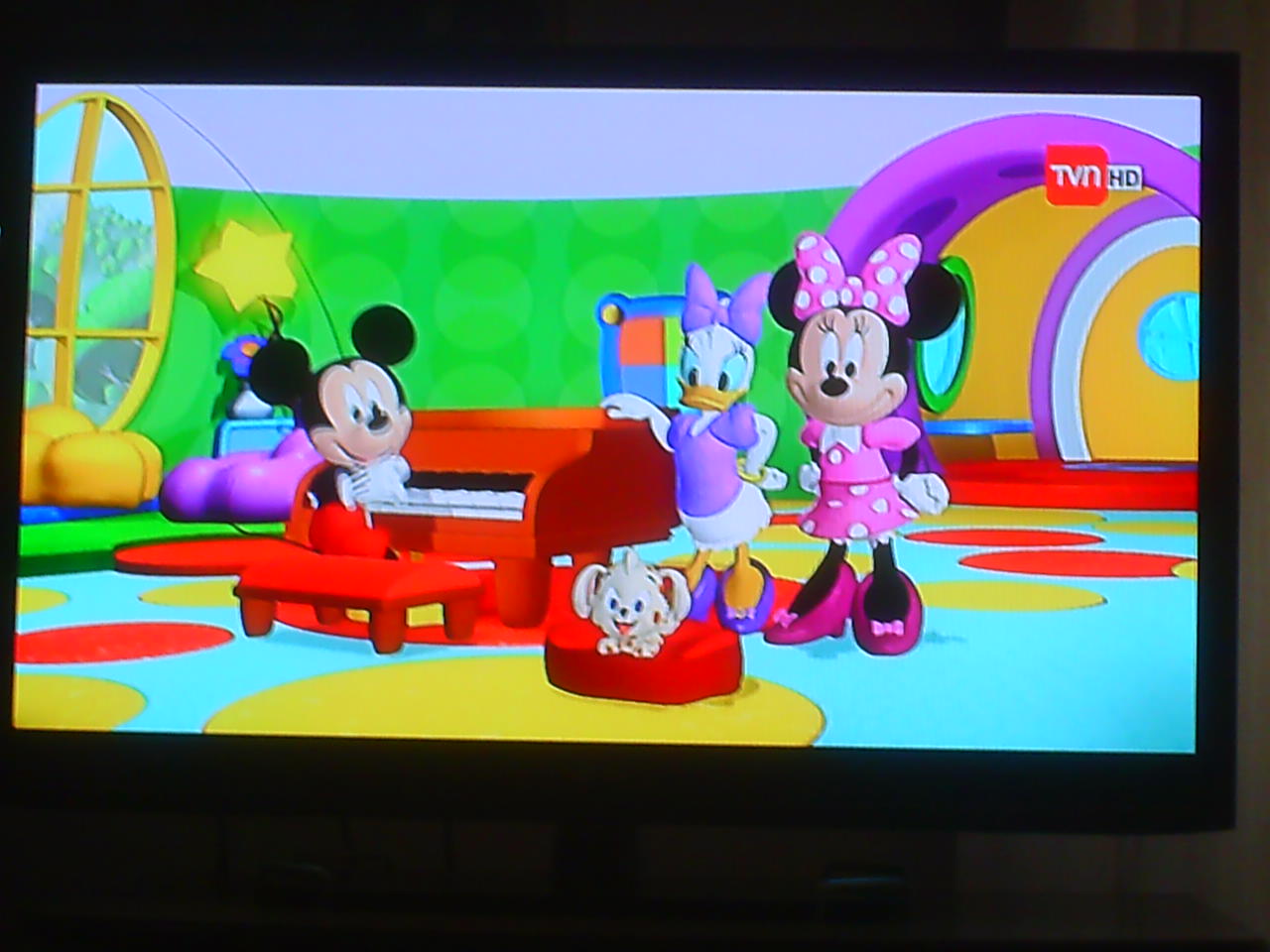The image is a photograph of a TV screen displaying a vibrant cartoon scene featuring Disney characters. The setting is a colorful room with large yellow and red polka dots on a white floor and green walls. In the scene, Mickey Mouse is seated at a bright red piano, wearing his iconic red shorts and white gloves. Minnie Mouse, adorned in a pink dress with a matching polka dot bow and purple shoes, stands beside him. Daisy Duck, dressed in purple with a bow on her head, stands nearby. A small puppy rests on a red pillow on the floor. The scene gives off a cheerful and inviting vibe. In the top right corner of the screen, the text "TVN HD" is visible. The photograph also captures glimpses of the darkened wall behind the TV and the surface on which the TV is placed, possibly a table or desk.